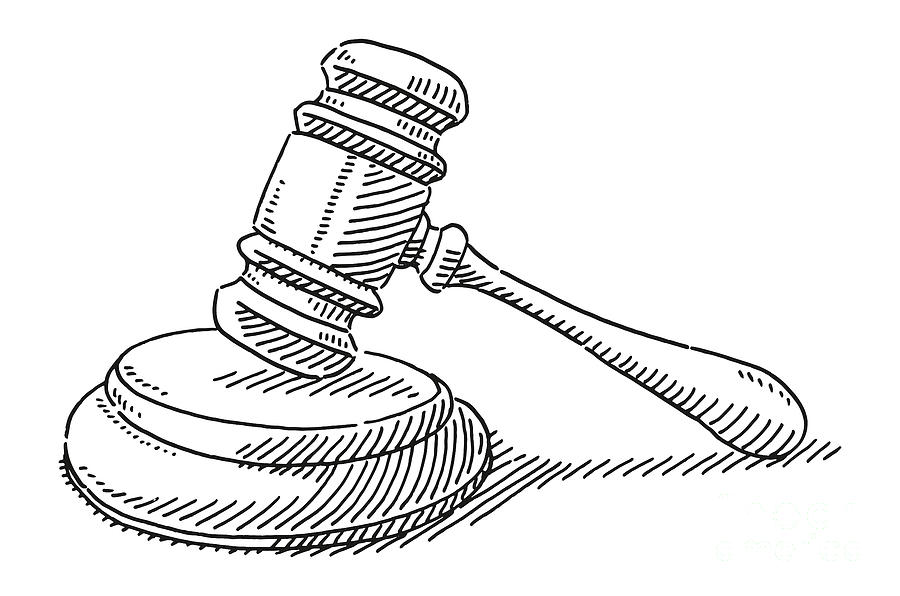This is a detailed black and white drawing on a white background, showcasing a judge's gavel and its stand. The illustration meticulously outlines the gavel's handle, which features finely drawn horizontal and vertical lines, enhancing its texture. The gavel's head is white with black ink detailing, including grooves that provide a sense of depth and dimension. The gavel itself is depicted leaning against the double-layered, circular stand, which has a thick base and a flat top layer where the gavel strikes. The entire image is intricately inked, combining detailed line work with layered shading, creating a visually striking representation of this courtroom symbol.